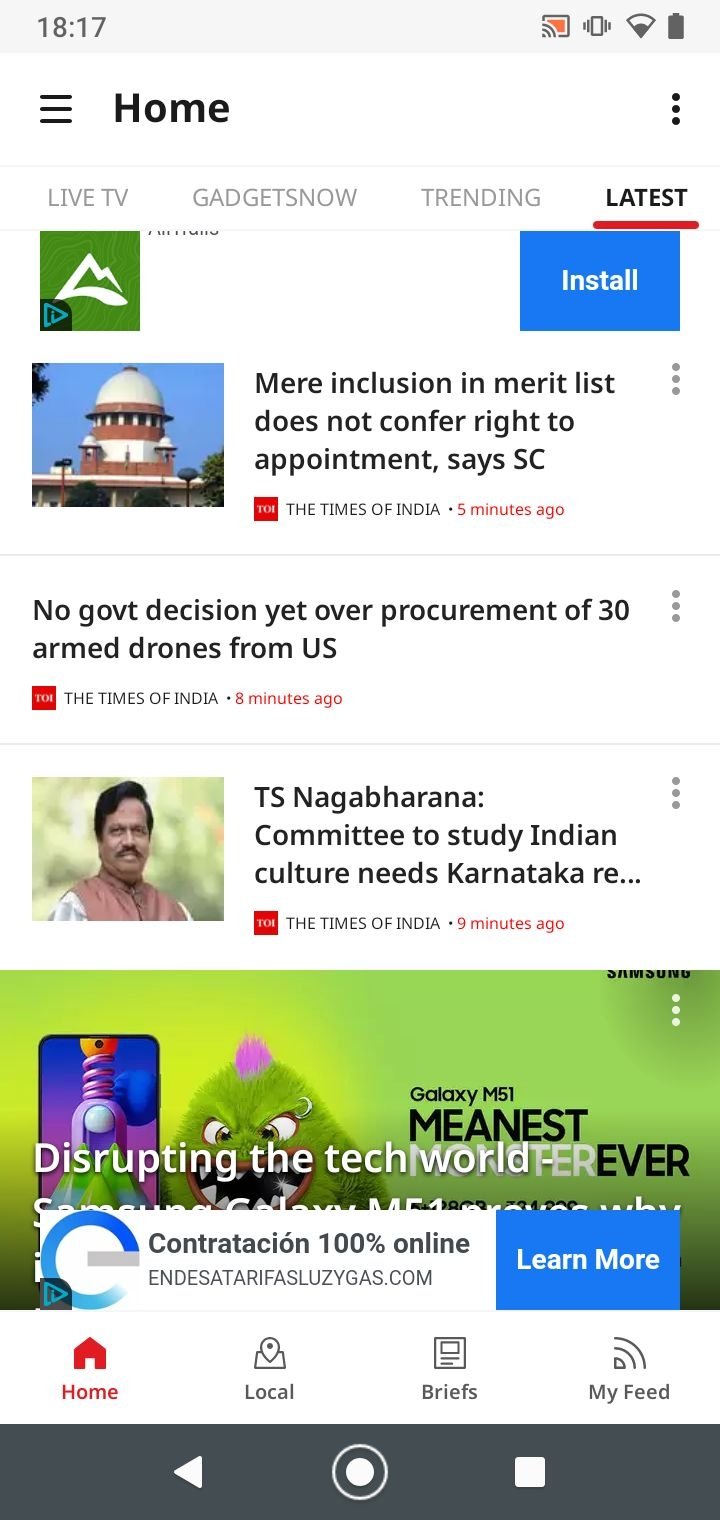This is a detailed screenshot from a smartphone display:

- **Top Section**:
  - The upper half-inch of the screen features a light grayish-blue background.
  - Across the top-right, a status bar shows the current time "8:17", a full battery icon, half Wi-Fi signal, vibration mode, and a screen share icon.

- **Middle Section**:
  - The screen background is white.
  - Below the time, three black horizontal lines appear, followed by the bold black text "Home".
  - On the right, three vertical black dots appear.
  - On the left, in a light black font, are the navigation options: "Live TV", "Gadgets Now", "Trending", and "Latest". The "Latest" option is bolded and underlined in red.
  - A green square with a white mountain outline icon is present on the left, next to a blue "Install" button in white letters.
  - Below, an image of a Capitol-like building with a blue sky is displayed. Adjacent to it, three bold black lines indicate text is present. The text below the image states the publication source and a red timestamp indicating how long ago it was published. On the right side, three vertical grey dots are visible.
  - There is a subsequent grey dividing line.
  - Beneath it, two lines inform about the publication source and timestamp, with three vertical dots on the side marking options.
  - Following another dividing line, an image of a man with a mustache and dark hair appears, indicating another news item or detail, followed by three lines of bold information specifying the source and timestamp, with three dots on the side.

- **Pop-up Section**:
  - The bottom portion includes a dark green background with a phone graphic and a small green monster with a purple mohawk, and next to it in green letters is "Disrupting the Tech World".
  - A white pop-up overlaps this section.

- **Bottom Section**:
  - A dark gray, almost black bar runs along the bottom inch of the screen. Red text indicates "Home" with "Local Briefs" near the user's feet in black text.
  - The familiar smartphone navigation buttons (a circle, a square, and a triangle) line the bottom edge.

This comprehensive image captures various UI elements, navigation options, and multiple layers of information, showcasing a typical vibrant, multi-tasking interface on a smartphone.